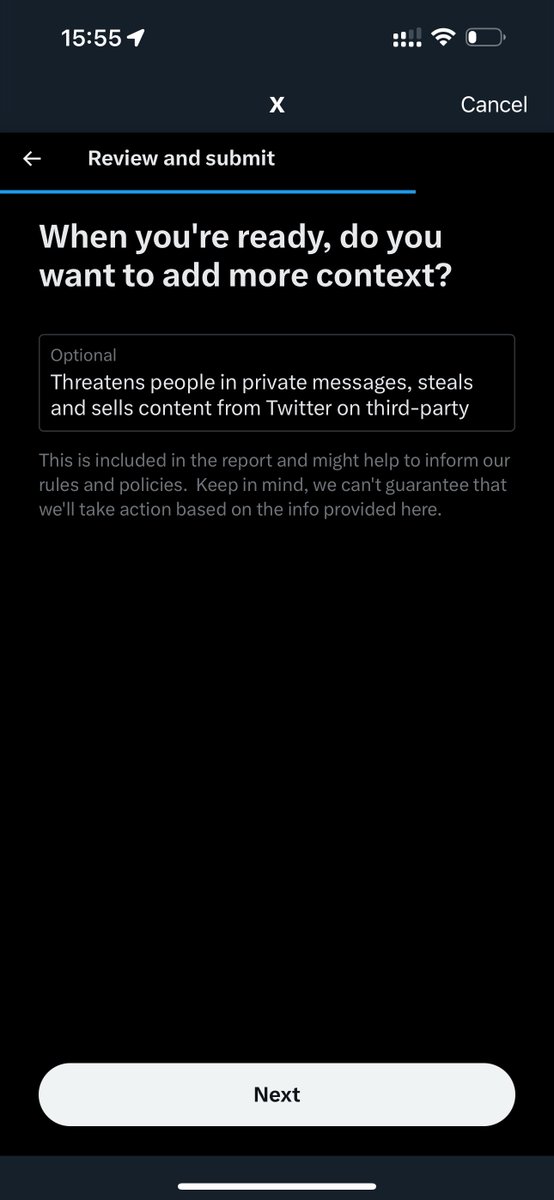This vertical image, likely captured on a smartphone, features a user interface screen with several distinct elements. At the very top, against a dull black background that almost appears gray in comparison to a darker adjacent black, is a horizontal rectangular bar. In the upper left corner of this bar, the military time "15:55" is displayed alongside a small location icon. On the right side of the bar, various status icons are visible, including signal strength, Wi-Fi, and battery life indicators.

Beneath this top bar, a centered white "X" is displayed with the word "Cancel" to its right. The background transitions to a solid, dark black with no visible texture or gradient. 

Below, a leftward-pointing white arrow accompanies the bold text "Review and submit." This section is separated by a blue line from the subsequent instructions. Following this, in larger bold white text, the prompt reads: "When you're ready, do you want to add more context?" Underneath, a light gray bordered box with the word "Optional" inside contains the text: "Threatens people in private messages, steals and sells content from Twitter on third-party."

Below this input field, a note states: "This is included in the report and might help to inform our rules and policies. Keep in mind, we can't guarantee that we'll take action based on the info provided here." At the very bottom of the screen, there is a button labeled "Next."